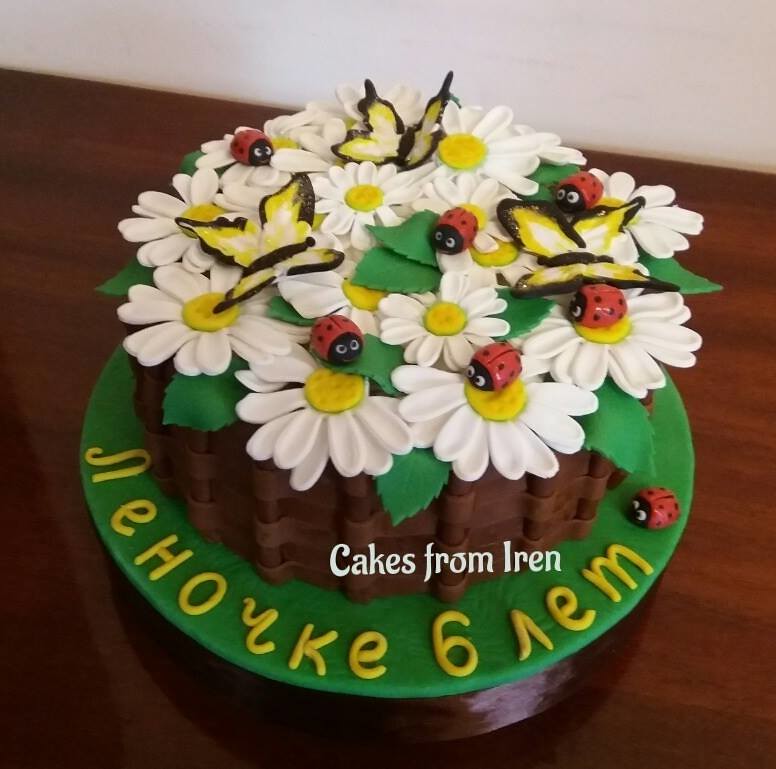The image is a square-shaped, color photograph, likely used as an advertisement for homemade cakes. Dominating the center of the photo is an ornately decorated cake, which sits on a brown hardwood surface. The cake's base is encircled by a green layer that resembles either a plate or decorative icing, giving the impression of grass. Above this green base, the cake itself appears to have a vertical, chocolatey brown center, possibly constructed with tubular-shaped cookies or chocolate layers designed to look like a basket weave or tree stump.

The top of the cake is lavishly adorned with numerous handmade white daisies, interspersed with green leaves, creating a lush floral scene. Scattered among the flowers are several small, detailed ladybugs with red backs, black dots, and black heads. Three large, visually striking butterflies, colored black, white, and yellow, are also perched among the flowers. Black text across the center of the cake reads "cakes from I-R-E-N," and there are additional yellow lettering in Cyrillic, suggesting it could be Russian or Ukrainian.

The background features a white wall at the top, providing a clean contrast that highlights the brown hardwood surface below, upon which the cake rests. Overall, the image captures a charming and detailed presentation, perfect for marketing the baker's homemade creations.